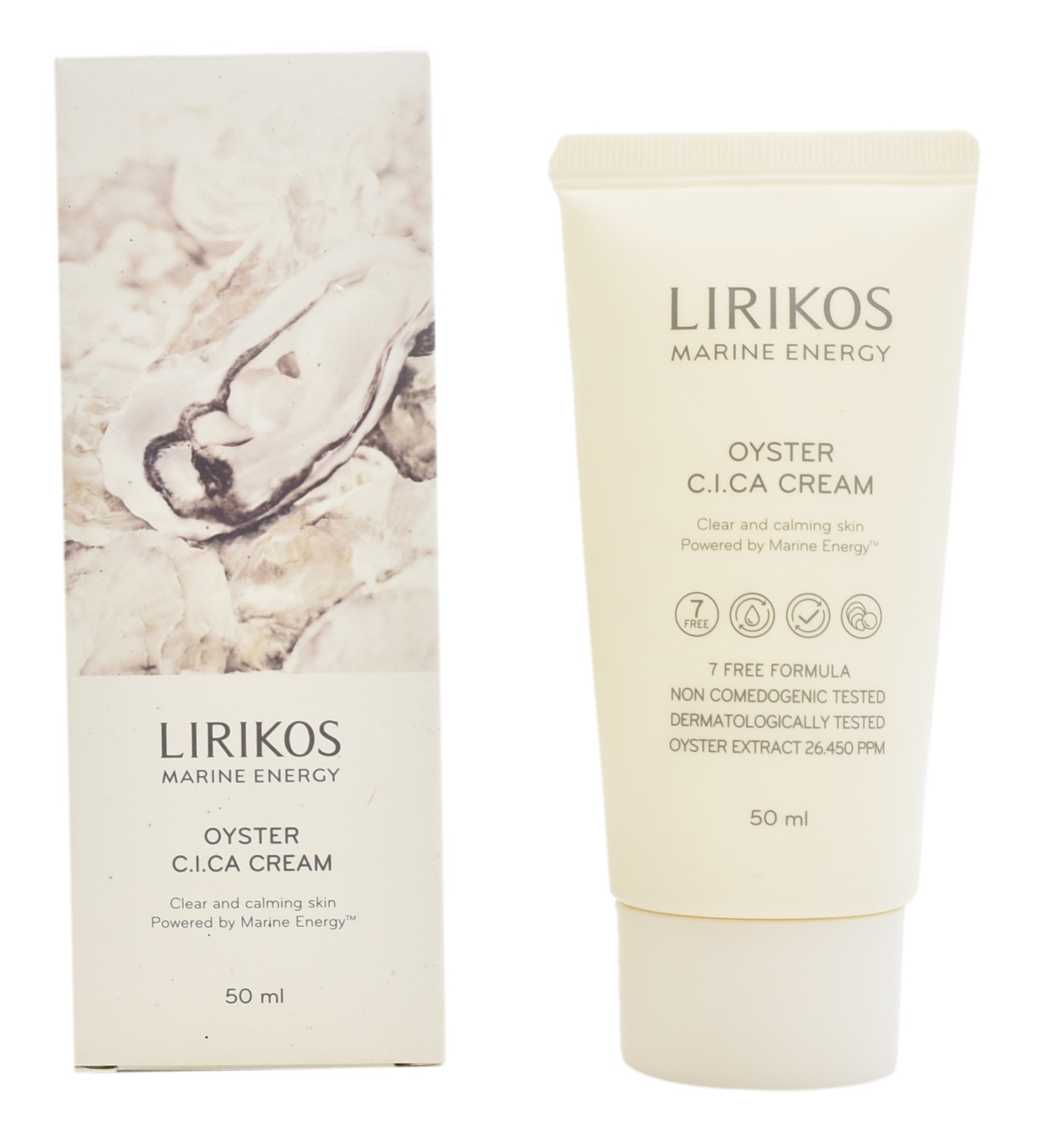This detailed product photo showcases the Lyrikos Marine Energy Oyster C-I-C-A Cream, designed to provide clear and calming skin powered by marine energy. The image consists of two main elements: on the left, there is a sleek rectangular box with a sophisticated color scheme of beige and gray tones. The top two-thirds of the box features a subtle black-and-white oyster image, and the bottom clearly states in gray letters, "Lyrikos Marine Energy Oyster C-I-C-A Cream." The description emphasizes its 50 ml capacity and highlights its clear and calming properties powered by marine energy, a trademarked statement.

On the right side, the actual product—a white, cream-colored squeeze tube—is displayed. The tube stands on its round, twist-off cap, indicating practical usability. It mirrors the box in terms of brand and product details, and adds additional information emphasizing sustainability and skin benefits. It features icons representing a 7-free formula, non-comedogenic testing, dermatological testing, and an indication of oyster extract concentration (26.450 ppm). The product has been carefully tested to ensure it doesn't clog pores, and its formula is ethically designed, likely with minimal to no animal testing.